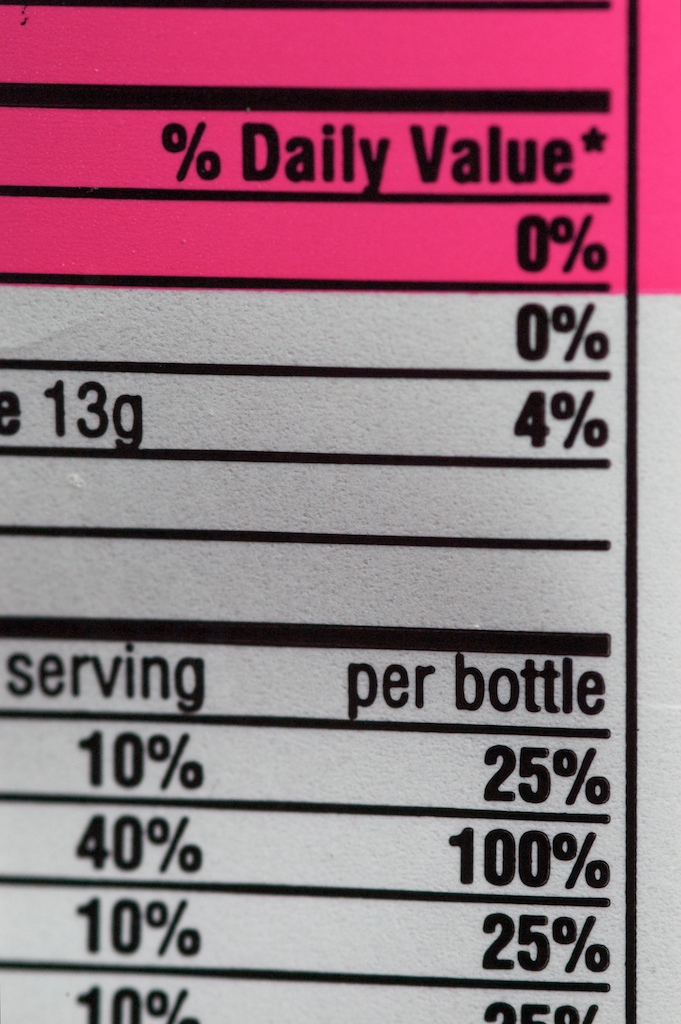The image features a Nutrition Facts label prominently displayed against a backdrop. The label is contained within a large rectangle and is printed in ink, which varies slightly in darkness, particularly along the first four white lines of text where there appear to be smudges of black dirt.

At the top, the label provides information broken down as follows:
- Percent Daily Value: 0%
- 'Y': 0%
- 13.4%
- Following are several percentage values: 10%, 24%, 20%, 100%, 10%, 25%, 10%, and 25%

The text is mostly white except for these percentage values. The caption "per bottle" is included, which likely refers to the serving size. The bottom portion of the label is predominantly white and cleaner compared to the top.

Overall, the smudges and dirt on the first four lines stand out against the relatively tidier lower section, giving the label an uneven appearance in terms of cleanness and print quality.